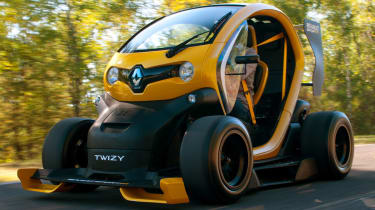A realistic photograph, horizontally oriented and taken during the daytime, features a unique, futuristic small vehicle prominently in the center on a paved surface. The vehicle, resembling a hybrid between a smart car and a golf cart, bears the name "Twizy" on its black front area in white letters. It is predominantly yellow with black accents, notably on the front. The design includes smooth tires and a rounded cockpit-like area with visible interior details such as a seat and seatbelt. This car, which has a top and a windshield but no side doors, appears to be driving on a highway. In the background, a sparse arrangement of trees can be seen.